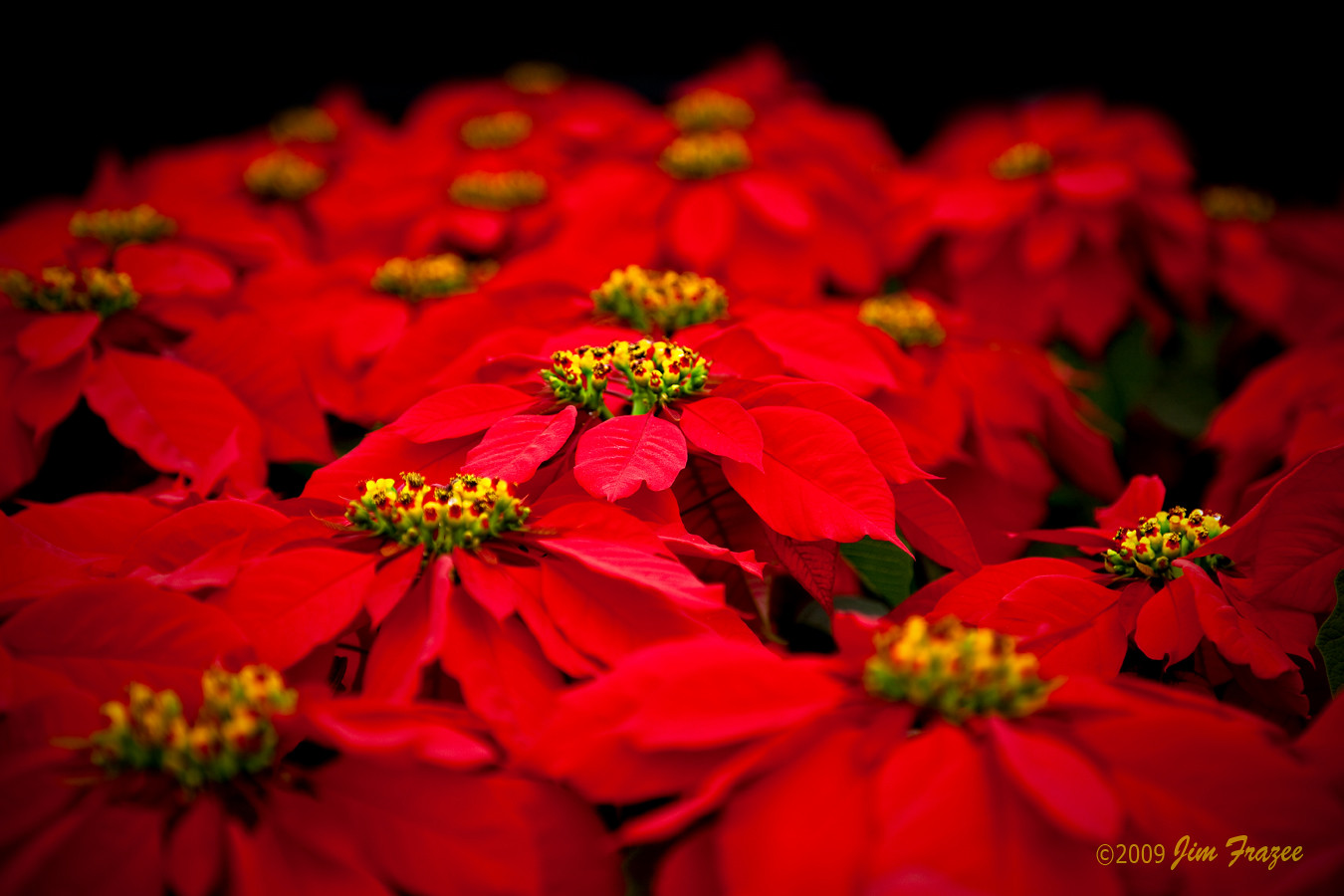A professionally taken photograph depicts an extensive array of vibrant poinsettia flowers, commonly associated with Christmas. The image is filled with numerous red-petaled flowers, each showcasing a yellow pollen center seated on green stems. The composition captures the flowers at eye level, with some in sharp focus towards the center and the foreground slightly blurred, giving a sense of depth. The background is predominantly dark, with subtle green leaves visible beneath the flower canopy, adding contrast to the vivid reds. In the bottom right corner, the text "© 2009 Jim Frazee" is elegantly printed in yellow, marking the image's copyright. The overall effect is a stunning, immersive visual of these iconic Christmas flowers extending into the distance.